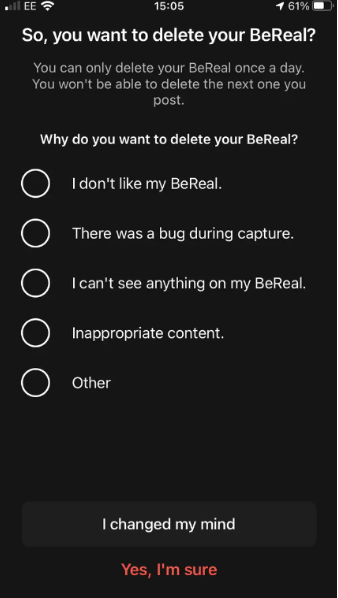The image is a screenshot from a smartphone displaying a social media application. At the top, there are standard smartphone icons: WiFi signal, a low battery indicator, and the time shown in military format as 15:05. The current battery life is at 61%. Below these indicators, a prompt with bold text asks, "So, you want to delete your BReel?" with "B" and "R" capitalized, followed by a question mark.

The prompt text is the largest on the screen, approximately 14-point font size and fully capitalized. Underneath this main question, a subtext in smaller but similarly styled font reads, "You can only delete your BReel once a day. You won't be able to delete the next one you post." This announcement suggests the functionality is related to a feature within a social media application.

Following this, there's another question, "Why do you want to delete it?" in a slightly brighter white font that matches the size of the subsequent multiple-choice options. The five options listed, none of which are selected, include:
1. I don't like my BReel
2. There was a bug during capture
3. I can't see anything on my BReel
4. Inappropriate content
5. Other

At the bottom of the screen, two action buttons are available: "I changed my mind" in white and "Yes, I'm sure" in red. The red button clearly represents confirmation for the deletion, emphasizing the finality of this action. All text is presented in reverse print with a black background and white lettering, ensuring clarity. The spacing between each multiple-choice option is uniform, contributing to a neat and organized visual layout.